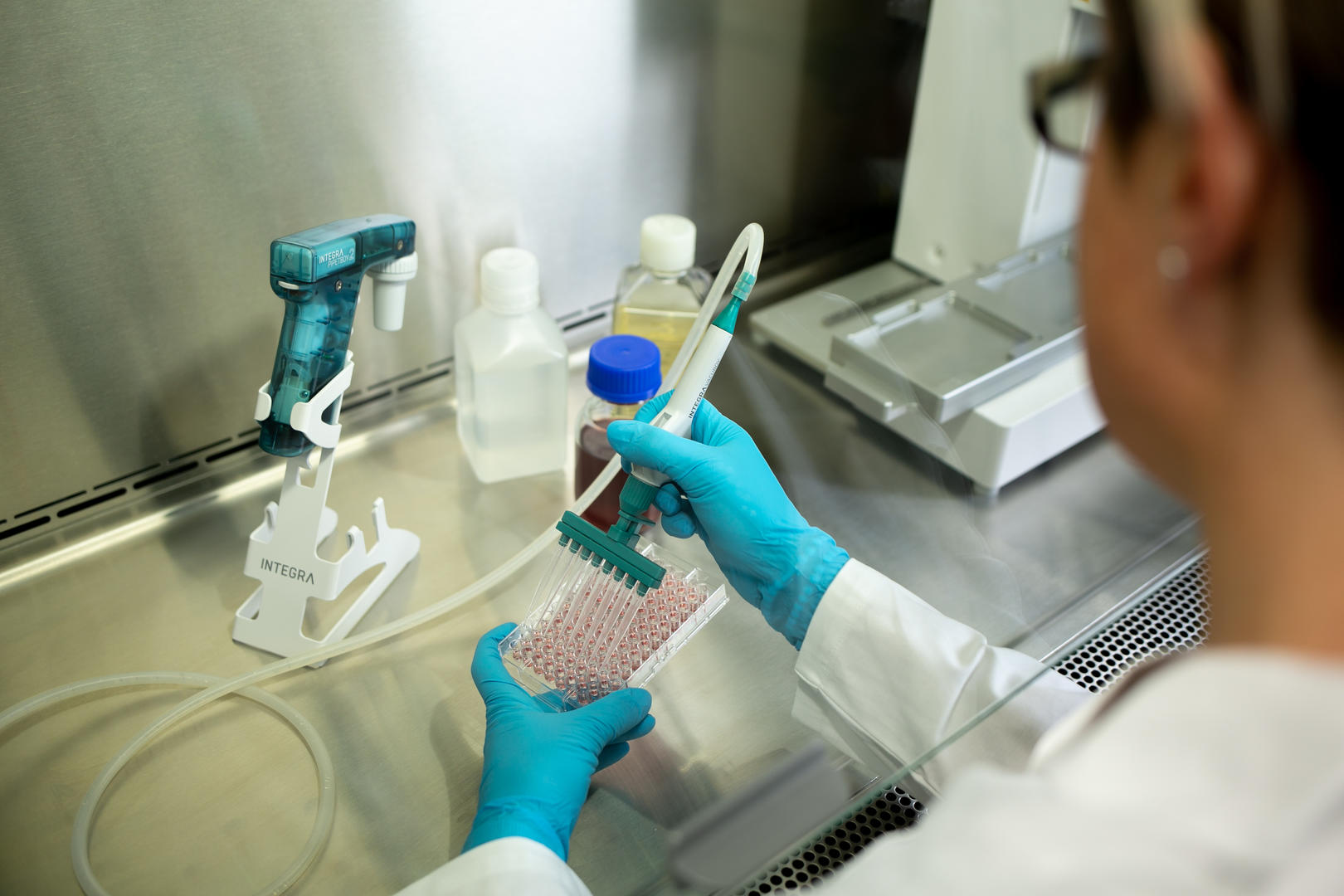The image captures a female scientist or technician working diligently in a laboratory setting. She is positioned on the right side of the frame, wearing a lab coat, light blue nitrile gloves, thin brown glasses, and a diamond earring. Her hair is tied up neatly. She is working on a stainless steel bench, illuminated by what appears to be a mixture of metal and glass surfaces. In her left hand, she is carefully holding a tray designed to hold multiple samples, possibly around 60. This tray contains small test tubes or wells meant for the experiment she is conducting. In her right hand, she uses a multi-channel pipetting device, equipped with eight pipettes, to simultaneously insert or extract liquid into/from the tray. This device is connected to a tube, which might be aiding in the liquid handling process. 

The bench is also populated with various bottles and equipment essential for laboratory tasks. Notably, there are three rectangular plastic bottles with large white caps, each filled with clear yellow or brownish-red liquids. Among the pieces of equipment, a striking blue, almost handgun-shaped device sits atop a stand, branded with the name Integra. Additionally, a scanning device resembling a soda gun in a white stand is visible on the table. The environment suggests meticulous scientific activity under stringent conditions, emphasizing the precision and care inherent in laboratory work.